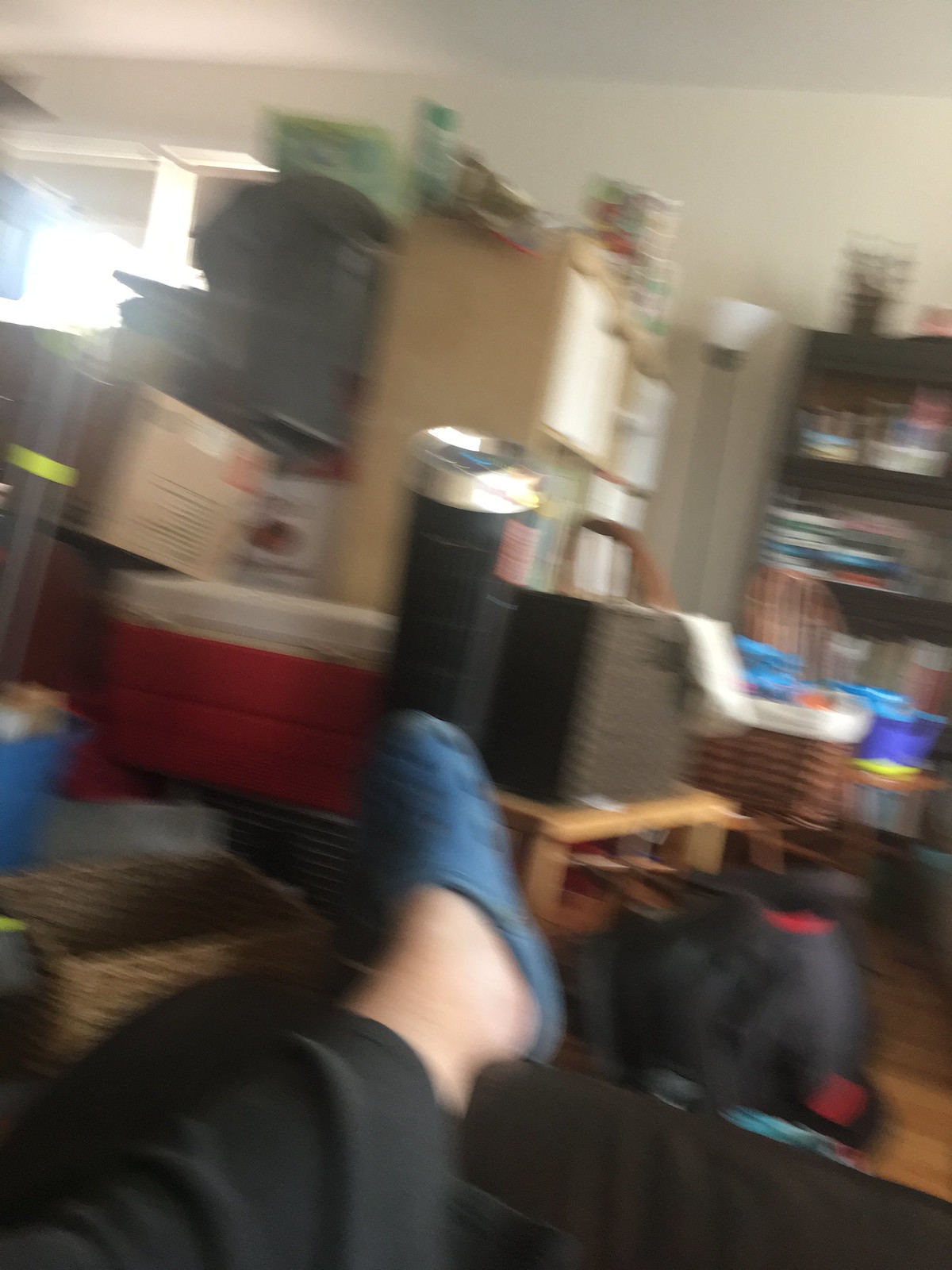The photograph is an extremely blurry and low-quality image taken from the viewpoint of the person capturing it, as evidenced by their left foot in the bottom left corner. The person, who appears to be Caucasian, is wearing loose black pants and blue Croc-style clog shoes. The cluttered background is indicative of a hoarder's home, with various items haphazardly stacked nearly to the ceiling, including cardboard boxes, baskets, and a red and white Igloo cooler. A black bookcase overflowing with items and a brown wicker basket are also visible. The chaotic scene takes place in what seems to be a living room with white walls and ceiling and a wood floor partially visible. In the upper left corner, there's a pathway illuminated by light, suggesting the presence of a window or an adjacent room. A tall torchiere lamp with a white shade is also discernible amidst the mess. The overall impression is one of extreme clutter and disorganization, making it difficult to distinguish specific details.